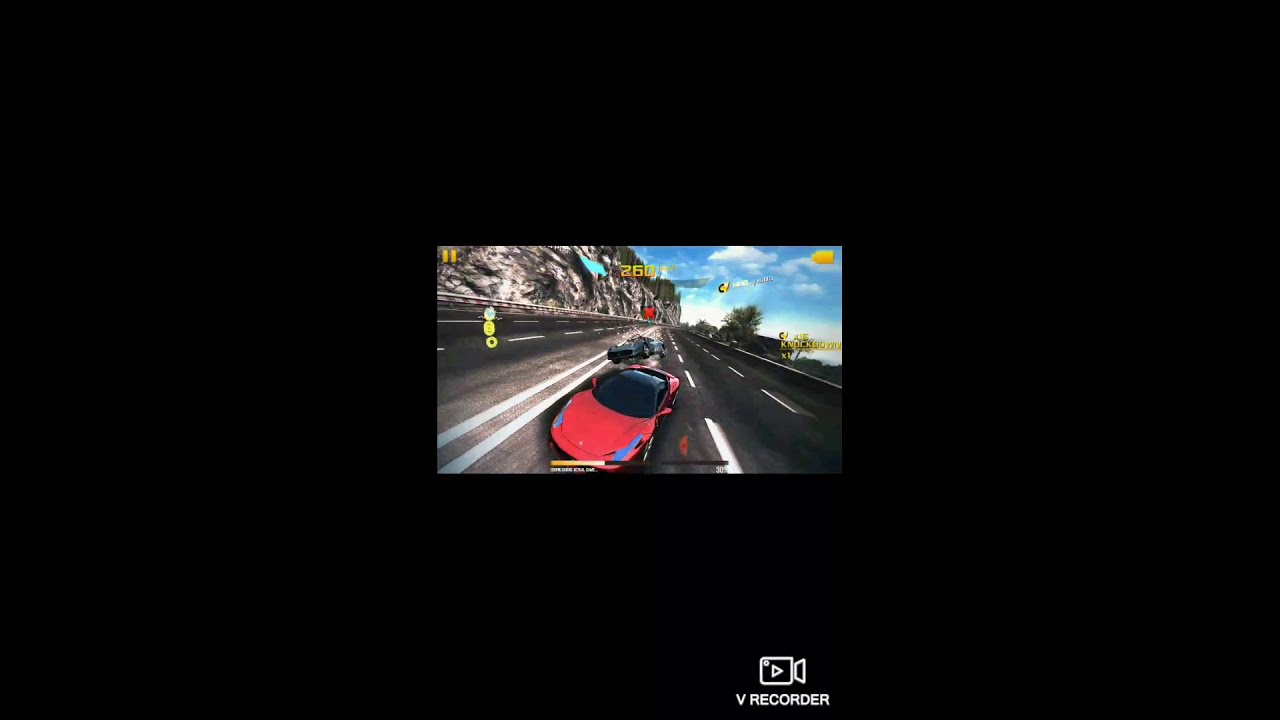The image is a screen grab from a high-speed racing video game, captured in a livestream indicated by the "V Recorder" icon and white text at the bottom center of the thick black border, which has pearlized specks adding a subtle shine. The main focus of the game is a red sports car, possibly a Ferrari, speeding towards the camera on a divided multi-lane highway with three lanes on each side separated by double white lines. The red car has a sleek black rooftop with tinted glass. Behind it, a gray or dark blue Porsche, which seems to have struck a guardrail, is in mid-crash, sending sparks flying. The background features a dramatic cliff face on the upper left, and to the upper right, a bright blue sky with scattered clouds enhances the racing scene. The screen also displays various numbers, scores, speeds, and controls, suggesting an intense and immersive gaming experience, although the graphics appear somewhat dated yet still moderately modern.